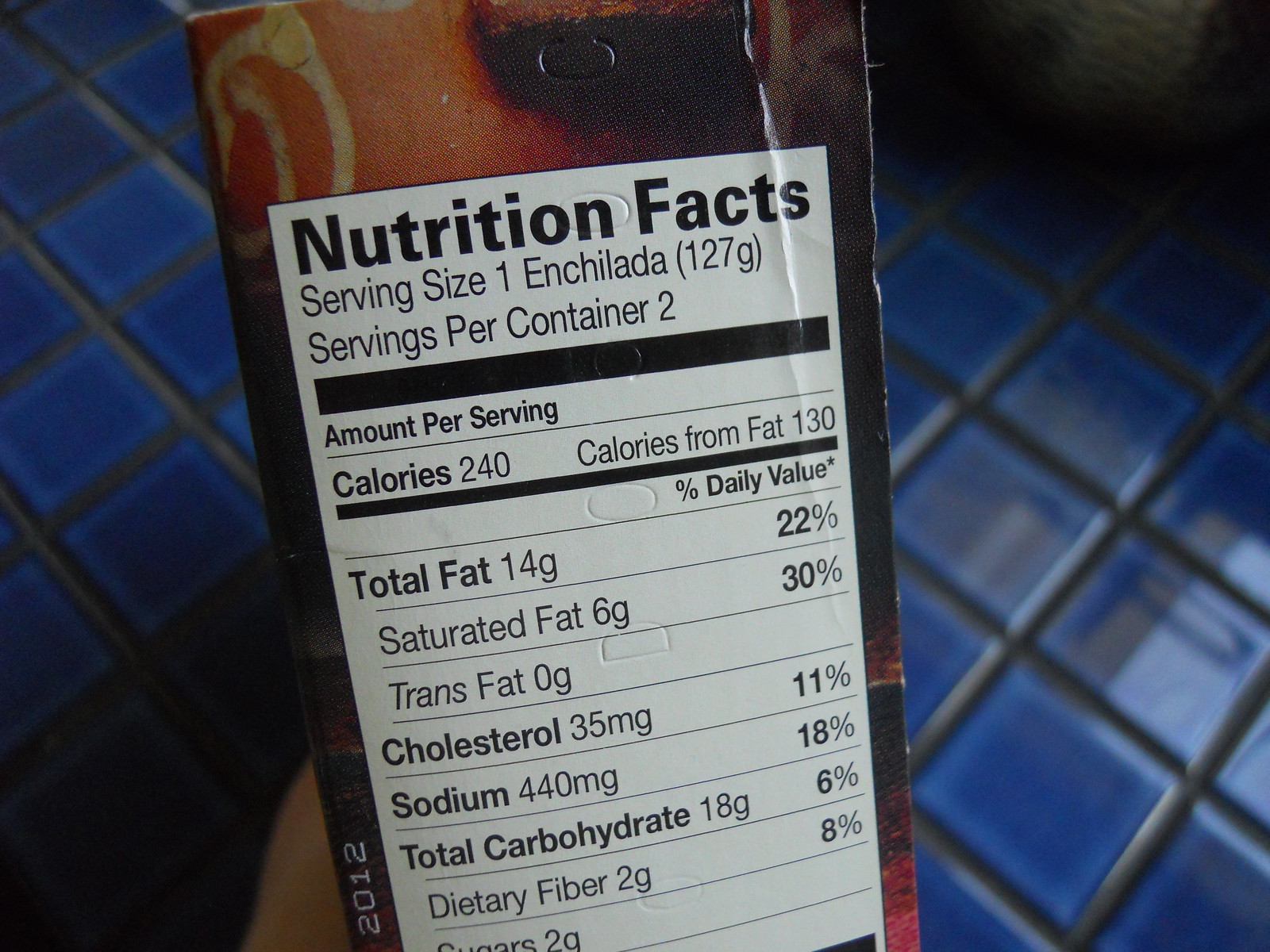A detailed close-up of the nutrition facts label found on the side panel of an enchilada box. The label specifies that each serving size is one enchilada, weighing 127 grams, with two servings per container. The nutritional information per serving includes: 240 calories, with 130 of those calories coming from fat. The total fat content is 14 grams, representing 22% of the daily recommended value, including 6 grams of saturated fat (30% DV) and 0 grams of trans fat. Cholesterol content is 35 milligrams (11% DV), sodium is 440 milligrams (18% DV), total carbohydrates are 18 grams (6% DV), and dietary fiber is 2 grams (8% DV). There is also a 2012 date printed on the left side of the nutrition label. The background features a tiled blue floor with perfectly square tiles, indicating that the photo was taken indoors. The packaging appears to be for an enchilada product, primarily brown in color, although only the side panel is visible and not the front or the product itself.